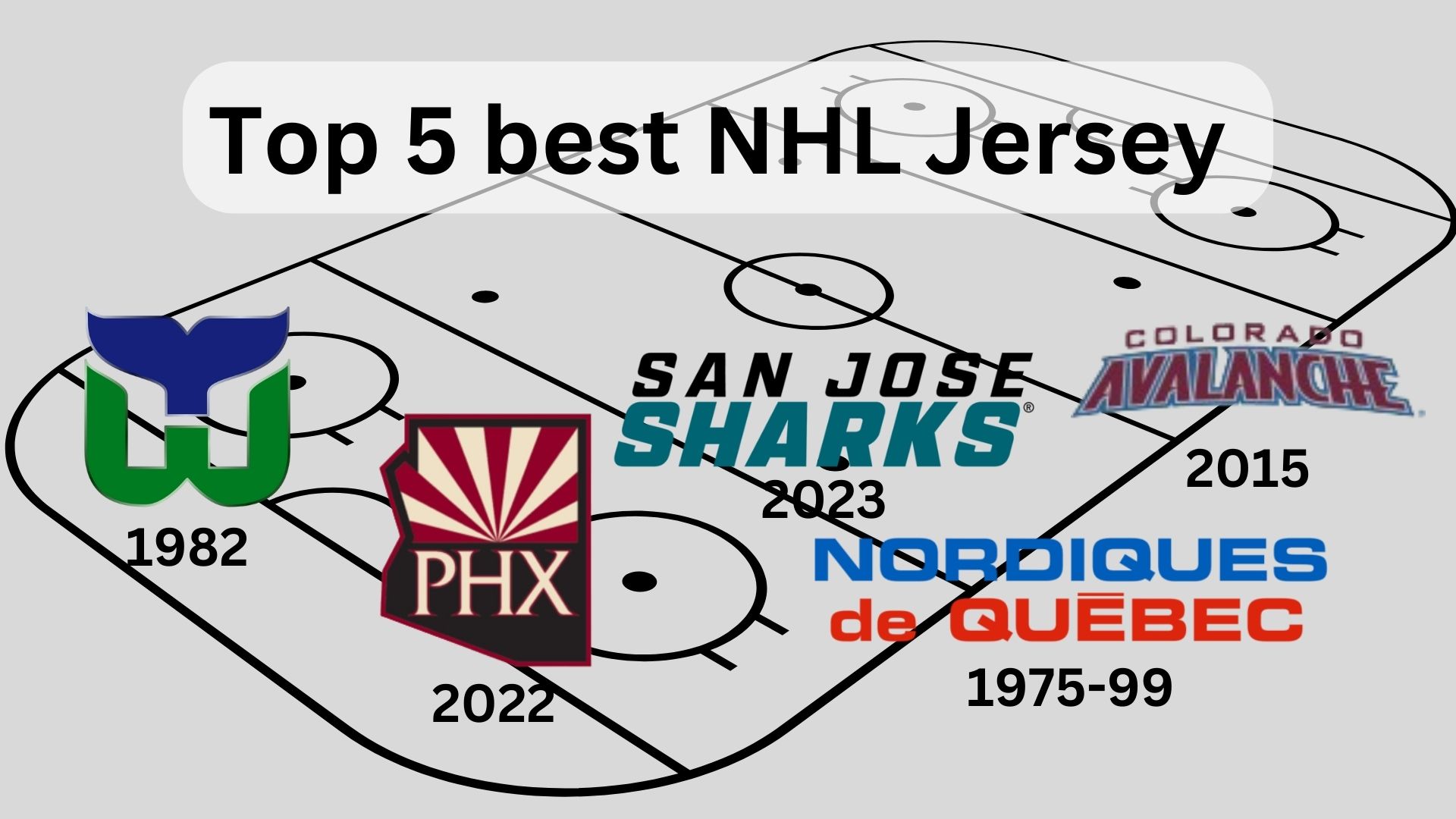This image serves as a promotional thumbnail designed for a blog or YouTube video titled "Top 5 Best NHL Jerseys." The background features a light gray bubble area at the top and a drawing of a typical black and white hockey rink, characterized by five circles and five lines. The main focus of the image is on the logos and dates of five NHL teams, aligned horizontally across the rink. 

From left to right, the image showcases:

1. A blue and green logo with a whale's tail emerging above a 'W', marked with the year 1982.
2. The state of Arizona with a rising sun pattern and the letters 'PHX', accompanied by the year 2022.
3. The logo of the San Jose Sharks, featuring the year 2023 below it.
4. The logo of the Nordiques de Quebec, with the years 1975-1999.
5. The Colorado Avalanche logo, marked with the year 2015. 

These elements are superimposed over the outline of a hockey rink, providing a visually engaging and detailed representation of the top five NHL jerseys according to the specified years.